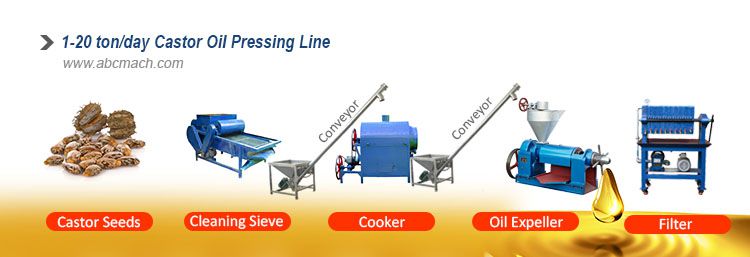The digital poster image is a detailed representation of the castor oil pressing line, structured in a clear sequence from left to right. In the top left corner, text in blue reads "1-20 tonne/day Castor Oil Pressing Line," followed by the website address "www.abcmach.com" in grey beneath it. Below, a row of five images illustrates the stages of castor oil production.

The process starts with the leftmost image, showing brown castor seeds labeled "Castor Seeds" underneath. Next to it is a blue machine with a flat base and a wheel, labeled "Cleaning Sieve," depicting the initial cleaning stage for the seeds. The third image shows a blue machine with adjacent grey components marked "Cooker," where the seeds are processed further. Following this, an "Oil Expeller" is depicted, a blue machine with some grey areas where oil is visibly dripping out. Finally, the rightmost image shows a "Filter," a blue apparatus on a metal base, indicating the final stage of filtering the oil.

The bottom part of the image features a yellow background, symbolizing oil, contrasting with the predominantly white background of the rest of the poster.